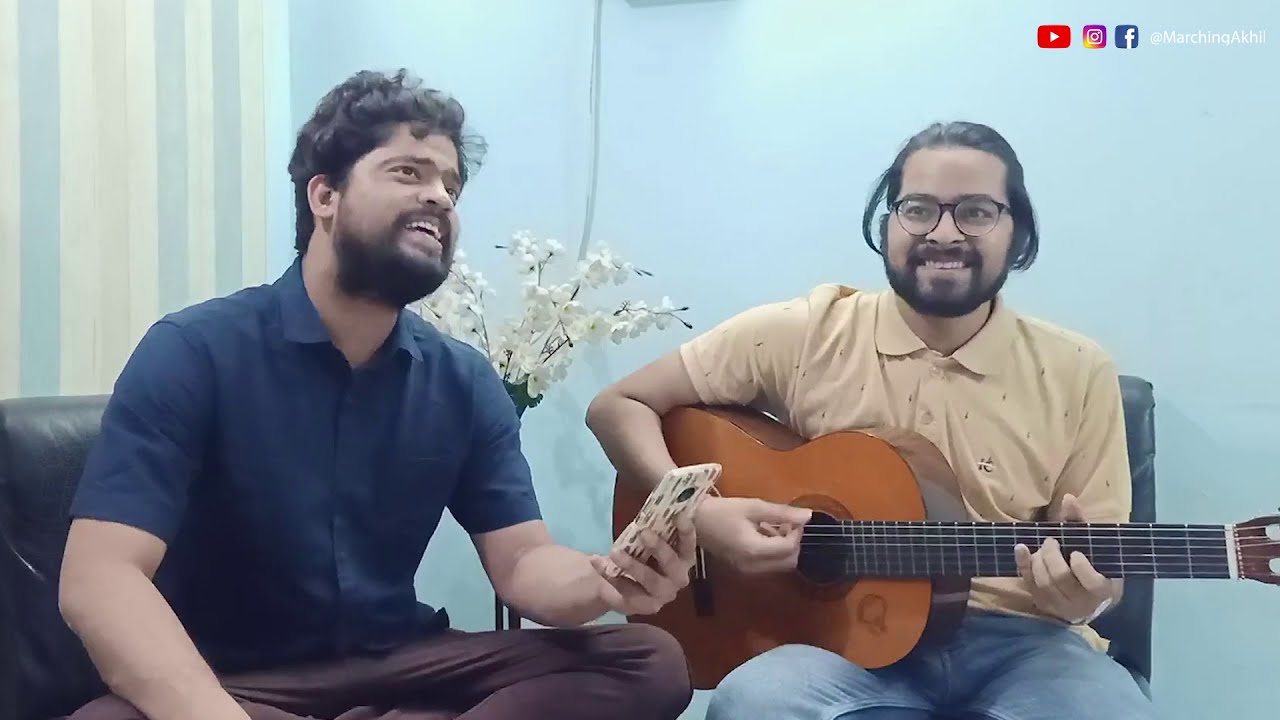In a cozy room with light blue walls and a corner adorned with striped paint, two men sit comfortably in chairs, both smiling and engaged in their activities. The man on the left is dressed in a blue short-sleeve button-up shirt and tan pants. He holds a cell phone in his left hand, which he extends slightly over his left knee, while his right hand rests on his leg. He has curly black hair, a beard, and a mustache, and his mouth is open as if he might be singing or speaking. Seated beside him, the man on the right is absorbed in playing a brown guitar, with his left hand positioned on the chords and his right hand strumming the strings. He wears a yellow polo shirt, blue jeans, and dark-framed glasses, showcasing his smile that reveals his top teeth. Behind them, a vase with white flowers adds a touch of nature to the scene. The upper right corner of the image features logos of Facebook, Instagram, and YouTube along with the text "Marching AKH." A cord is partly visible behind the flowers, adding to the casual ambiance of the setting.